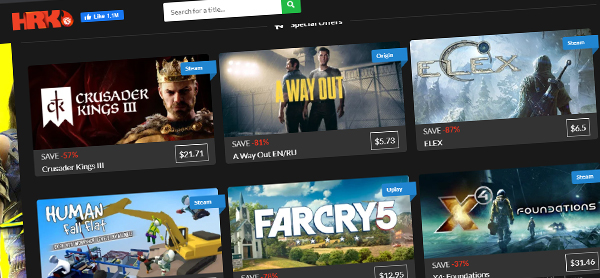A screenshot captures an angled view of a screen, possibly an advertisement or a photograph taken of a display. In the upper left corner, the HRK logo is prominently featured, accompanied by a graphic depicting a fire. The image also displays a significant social engagement with over 1.5 million likes. Below this, there's a search function highlighted with a green button. 

The content primarily shows a marketplace for purchasing movies, shows, or games, all set against a gray background with rectangular tiles. Titles include "Crusader Kings II" and "Crusader Kings III," each illustrated with a protagonist donning a crown. "Crusader Kings III" is priced at $21.71. Another prominent title is "A Way Out" priced at $5.73, showing two characters standing in a warehouse. 

To the right, there's an image of a warrior with a sword on his back and a hood, set against a snowy landscape, priced at $6.50. Nearby, a game titled "Human: Fall Flat Construction Site" reveals simple, minimalistic graphics. Another game, "Far Cry 5," is listed at $12.95. Finally, there's "X Foundation" priced at $31.46, visible on the far right of the display.